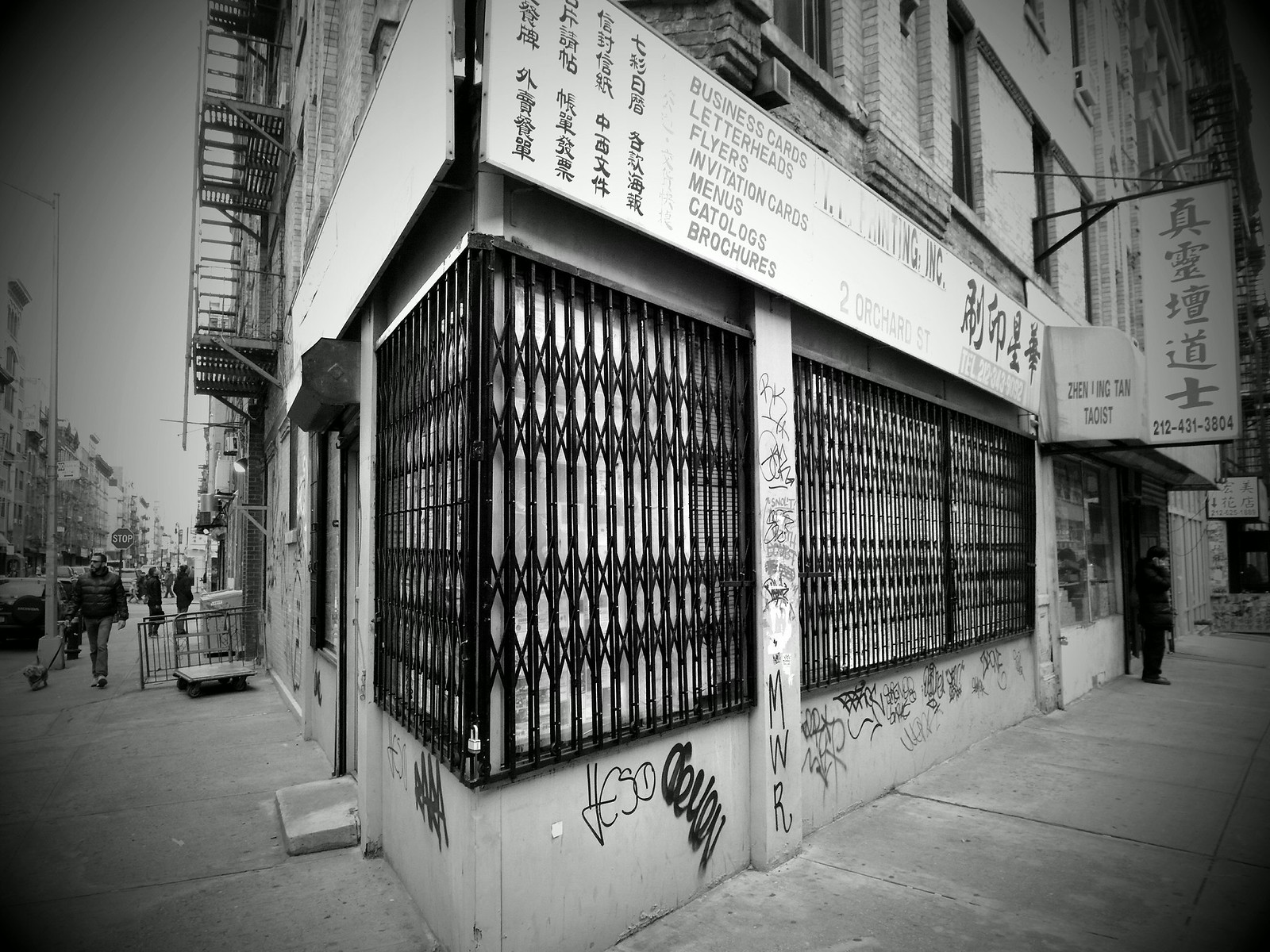This black and white photograph captures a busy daytime scene at a corner in New York City's Chinatown. The image prominently features a building on the corner, which is partially boarded up and secured with wrought iron bars on the windows. The lower part of the building façade is covered in graffiti running from left to right. 

An awning with signage in both English and Chinese hangs above, reading "Zen Jing Tan Taoist" and promoting various printing services including business cards, letterheads, flyers, invitation cards, menus, catalogs, and brochures. The phone number 212-431-3804 is clearly visible. Above the awning, there's additional Chinese writing.

On the left-hand side of the image, the sidewalk stretches back into the distance. Three people are visible; one person is walking a dog towards the camera, while two other individuals walk away. Further back, more pedestrians can be seen along with a stop sign. There’s a fire escape and a small wooden trolley adjacent to the sidewalk. 

On the right-hand side, a person stands under the awning, possibly speaking on a phone. The photo's monochromatic nature emphasizes the urban texture and details, making the presence of graffiti and the building’s closed, gated state even more pronounced.